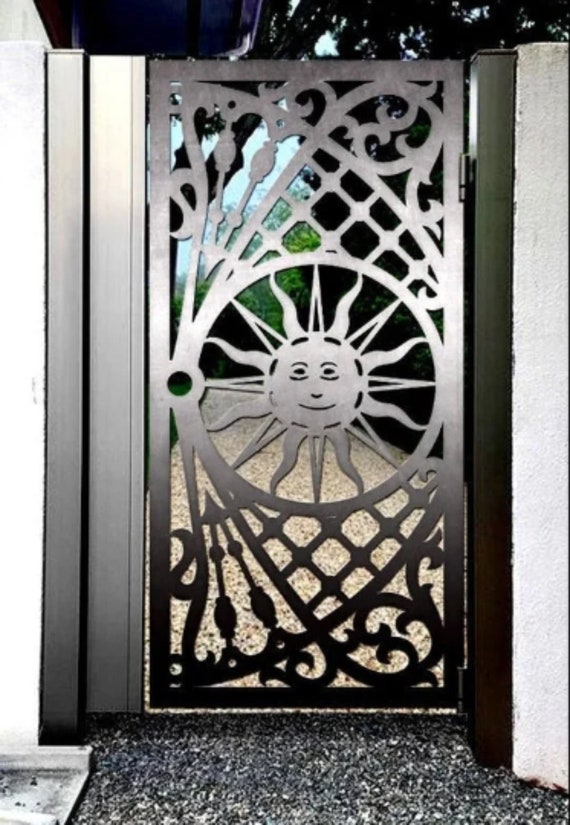The image captures a detailed view of a metal gate door, likely made of iron, featuring an intricate design cut by a 2D plasma cutter. The door showcases a prominent pattern, including a circle with a sun at its center, smiling down amidst swirling arrows, leafy motifs, and various curves. This circle, acting as a handle, is situated slightly off-center to the left, while two metal hinges are visible on the right, allowing the door to swing open. The door’s frame, sharing a similar metal texture, exudes a brownish hue accented with white reflections, blending seamlessly with its surroundings. 

The door opens to reveal a lush outdoor area with green trees and brown branches visible beyond. The surrounding walls inside the doorway are stark white, contrasting the door's dark, intricate design. Below, the ground is covered by an aggregate rock pathway, featuring shades of brown, white, and gray, complemented by what appears to be a white water runoff with dirt in the lower-left corner. The light source behind the camera illuminates the door's face, enhancing the detailed patterns and adding depth to the overall scene.